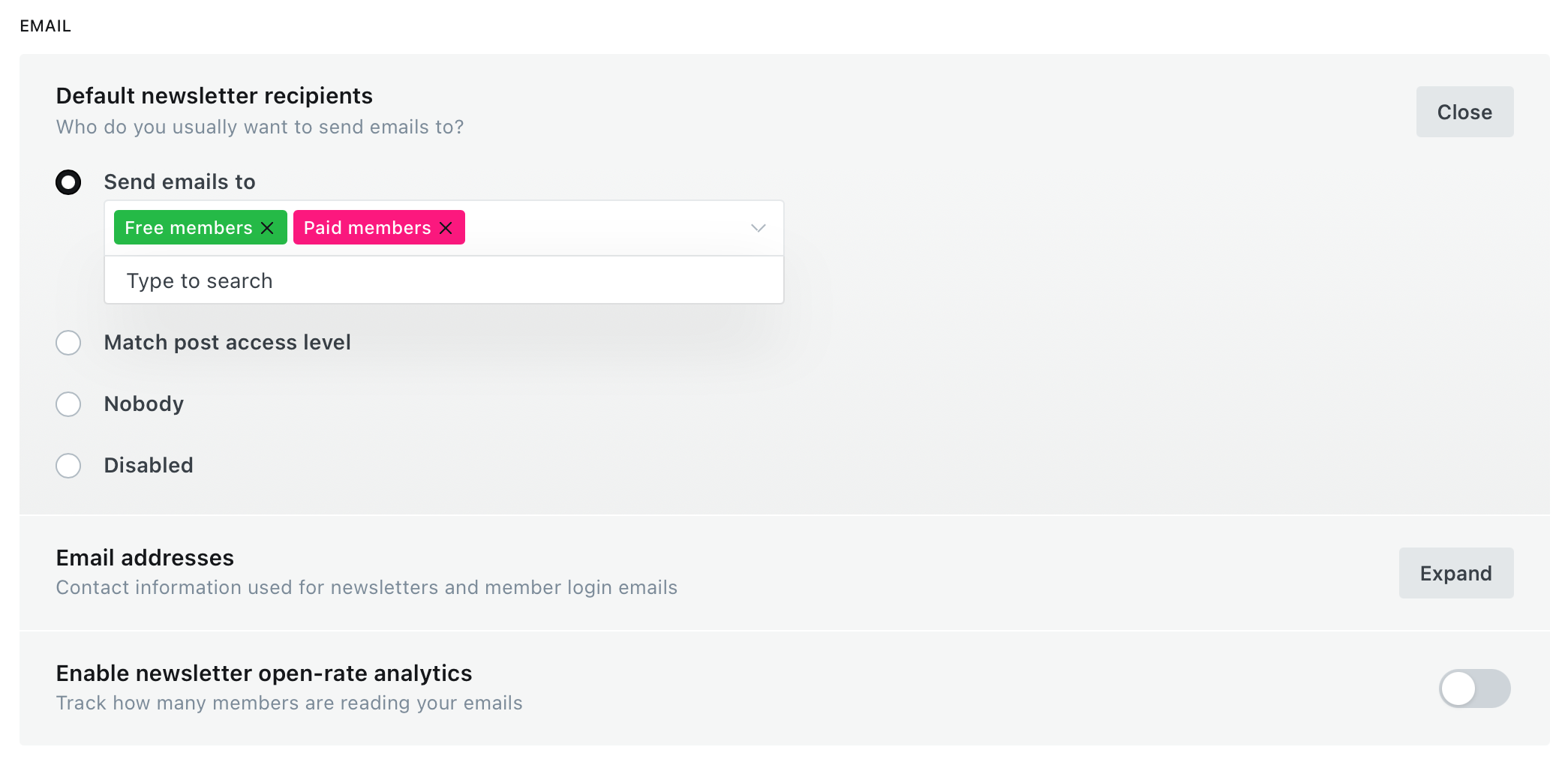Here is a cleaned-up and detailed caption for the described image:

---

This screenshot captures the interface of an email client, specifically a settings panel for managing newsletter recipients. At the top-right corner, there's a close button set against a light gray background. Below it, on the right side, is an expand button located just above a horizontal slider bar.

The main panel is titled "Default Newsletter Recipients," with the primary section showcasing two highlighted categories for email recipients: a green icon labeled "Free Members" and a pink icon labeled "Paid Members." Next to each icon, there are 'X' buttons that allow users to remove recipients from the list.

Above these categories is a search bar labeled "Type to search," which lets users filter recipient types. Below the recipient section, there is a series of unselected open circles with labels like "Match Post," "Access Level," and "Nobody Disabled," which appear to offer additional filtering options.

Further down, there's a section titled "Email Addresses," which references contact information used for newsletters and member log-ins, accompanied by an expand button on the right. Another segment titled "Enable Newsletters Open Rate Analytics" is shown, with a toggle switch set to the left in the 'Off' position, indicating that tracking how many members are reading the emails is currently disabled.

The entire recipient selection area sits on a white field and is accented by a pronounced drop shadow, giving it a floating appearance and distinguishing it from the three options listed below.

---

This detailed caption provides a comprehensive description of the email client's interface, highlighting various features and settings available to the user.